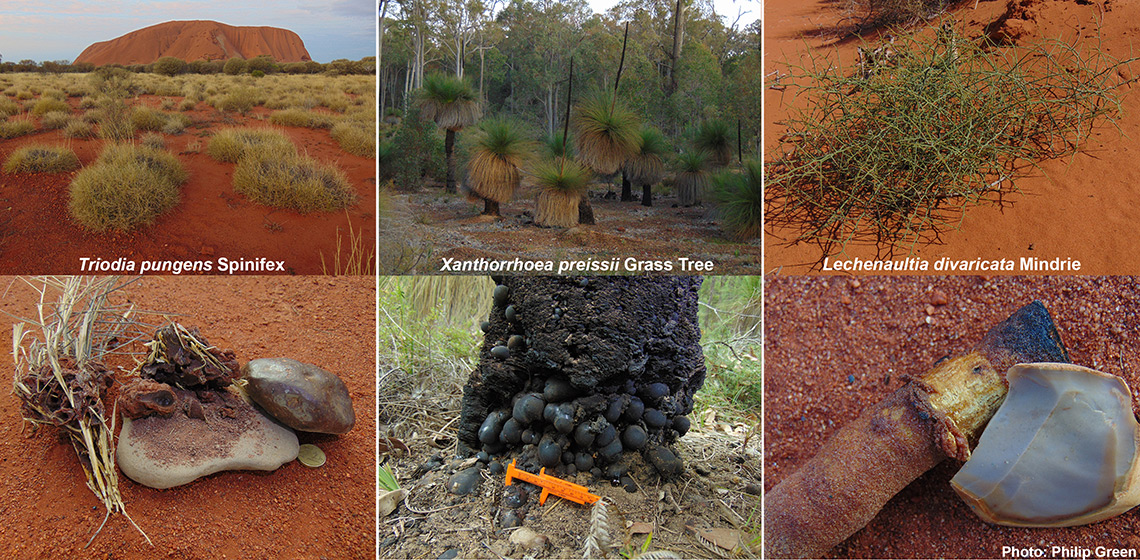This six-paneled image compilation showcases diverse natural scenes, each panel highlighting unique landscapes and plant life. 

In the top left, there's a reddish desert expanse with clusters of greenish-beige grass and distant brown-red hills, captioned "Schrodinger Pungent Spin Effects." Moving right, the second panel features a verdant forest with trees resembling palm trees—captioned "Xanthohoria Priscia Grass Tree." The third top panel presents another desert scene with tumbleweeds, captioned "Lechonotikola Devaritikamenindri."

The bottom left panel depicts a dried-out orange plant amidst rugged rocks and branches. The central bottom image features a dark plant with a mysterious, almost mossy texture, complemented by a small orange ruler in the foreground. The bottom right panel displays a simple scene of a branch lying next to a rock on reddish soil.

Each image, arranged in two rows of three, captures the plants in their natural habitats, styled in Photographic Representationalism Realism. Photo credit: Philip Green.